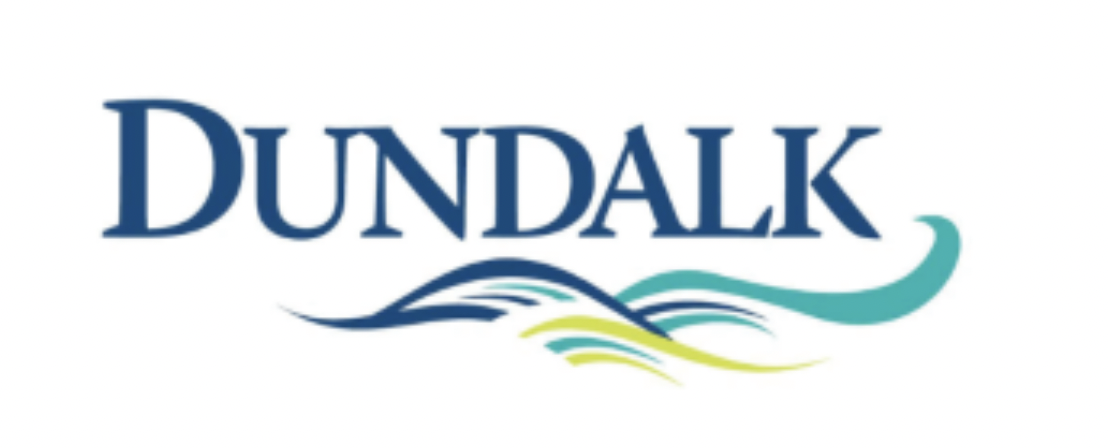The image features a simplistic yet meaningful logo on a completely white background. Centered and bold, the dark blue text "DUNDALK" is spelled out in all capital letters, with the 'D' slightly larger than the rest. Below the text, an array of wavy lines in varying colors — dark blue, teal (or seafoam green), and yellow-green — create a visual impression of waves, suggesting a nautical theme possibly related to a lake, beach, or the ocean. The dark blue wave has a unique, branching pattern, with one section swooping down, then up, and down again, while another branch moves upwards and back down, adding a sense of motion. The teal waves feature multiple inflection points and shorter curves, reminiscent of the shape of eyebrows, adding to the dynamic feel. This logo likely represents a business or product connected to water or maritime activities.